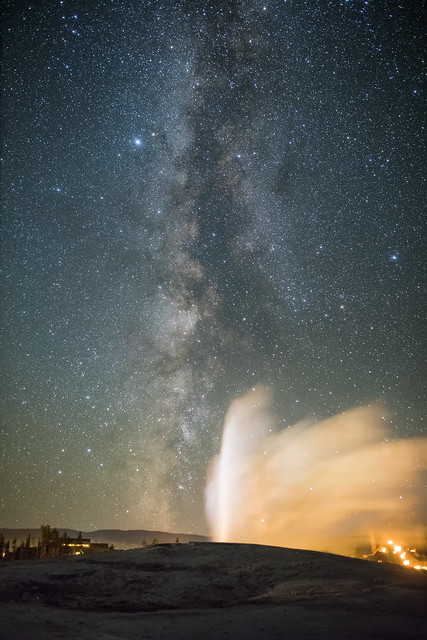The image showcases a stunning night sky densely populated with stars, where pathways resembling a nebula or foggy textures extend across the clear expanse. In the portrait-oriented image, the upper section vividly portrays a gradient sky that darkens at the top and fades into a lighter blue as it descends. Amidst this celestial display, a darker central area contrasts with the star-filled regions on either side.

The bottom part of the image reveals a rural or desert-like landscape featuring a prominent, spouting geyser spraying water high into the air. This vibrant scene is split into a lit building on the left and additional lights on the right side. The lower eighth also includes a small hill, beyond which the upper portion of the geyser dramatically shoots water to the right, punctuating the serene yet dynamic night tableau.